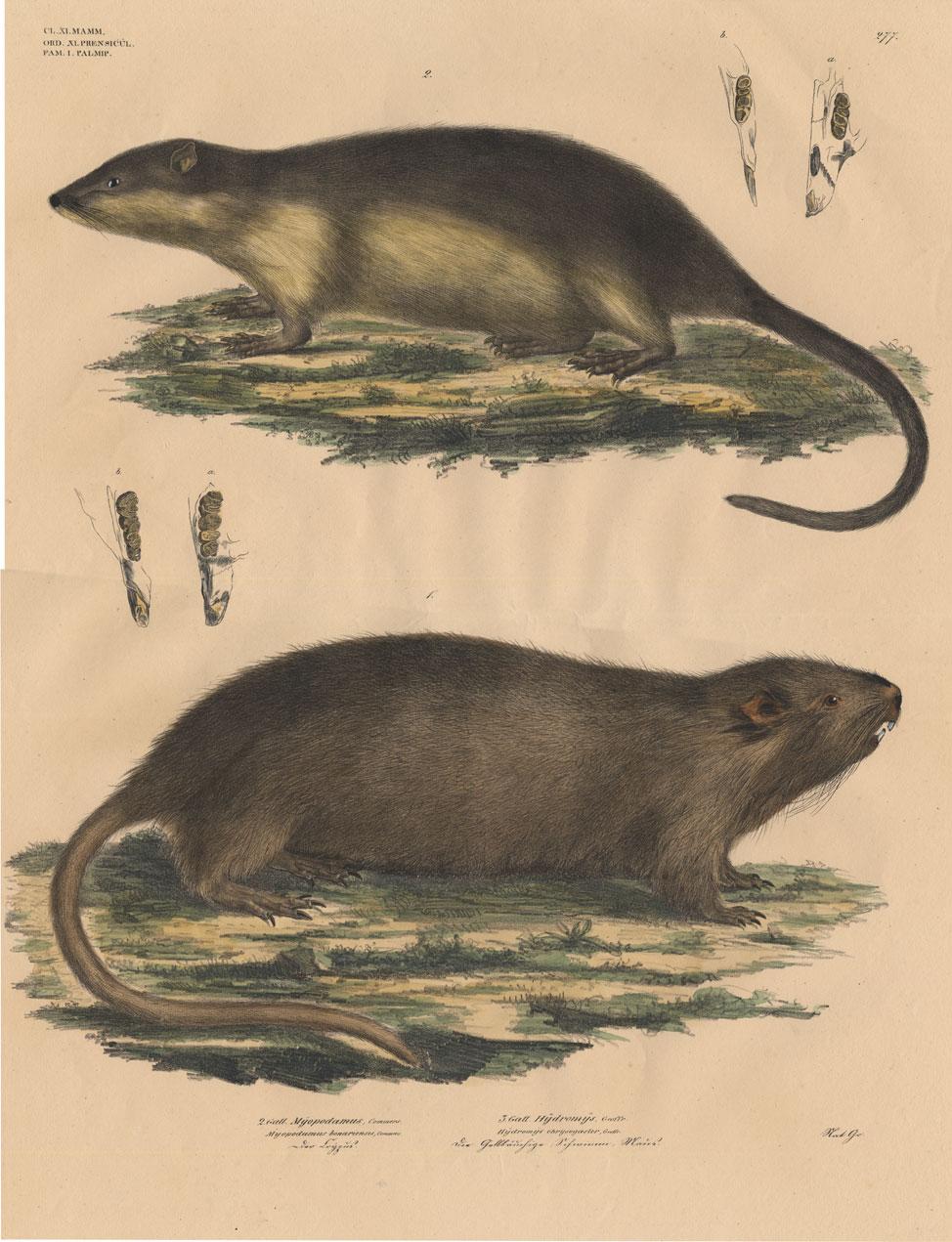The image depicts two illustrations of a large rodent-like animal, resembling a cross between a rat and a beaver, each set against a white background with some writing and dots throughout. The upper illustration shows the animal facing left, with a triangular-shaped head, closed mouth, long, thick body, short legs, and a long, pointy tail. The lower illustration portrays the animal facing right, with its mouth open to reveal sharp, white teeth on both the upper and lower jaws. The animal is depicted standing on a small piece of land covered with green plants and brown soil, indicating its natural habitat. The rodent has a grayish color with a hint of green, suggesting it might be quite strong and well-suited for its environment.